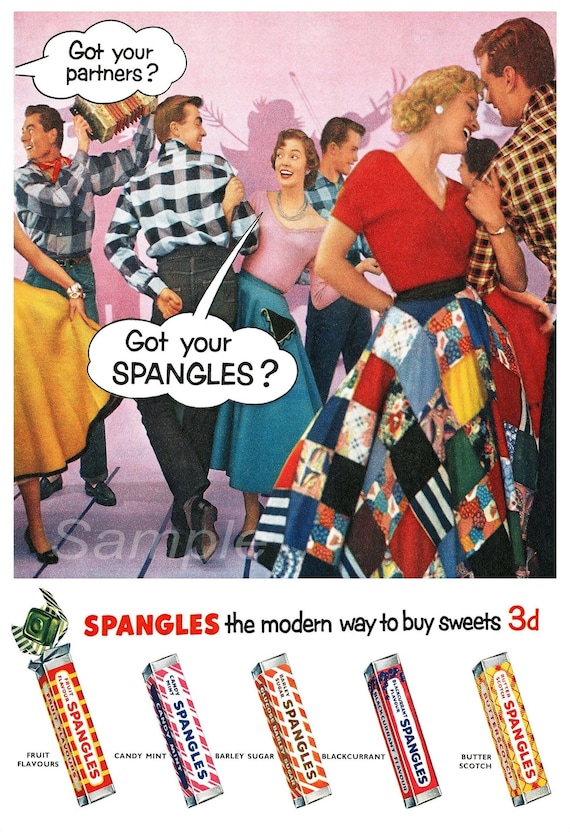This vintage advertisement poster, likely from the 1950s, features a lively square dance scene with teenagers dressed in period-appropriate attire. The young men sport 1950s pompadour hairstyles, with some wearing plaid flannel shirts and ascots, while the girls are in long dresses reminiscent of the era, including one with a quilt-like design. They appear to be dancing, with the shadow of a violinist in the background adding to the dynamic atmosphere. The poster contains playful text bubbles with lines such as "Got your partners?" and "Got your Spangles?" 

At the bottom of the poster, the product being advertised is Spangles, a type of hard candy that comes in a rectangular, gum-like package. The poster promotes Spangles as "the modern way to buy sweets," with flavors including fruit, candy mint, barley sugar, blackcurrant, and butterscotch. The slogan and packaging suggest a novel confectionery experience, and the term "3D" appears, hinting at a promotional trend or price, although its exact meaning remains unclear. This colorful and energetic advertisement captures the charm and style of mid-20th-century culture.